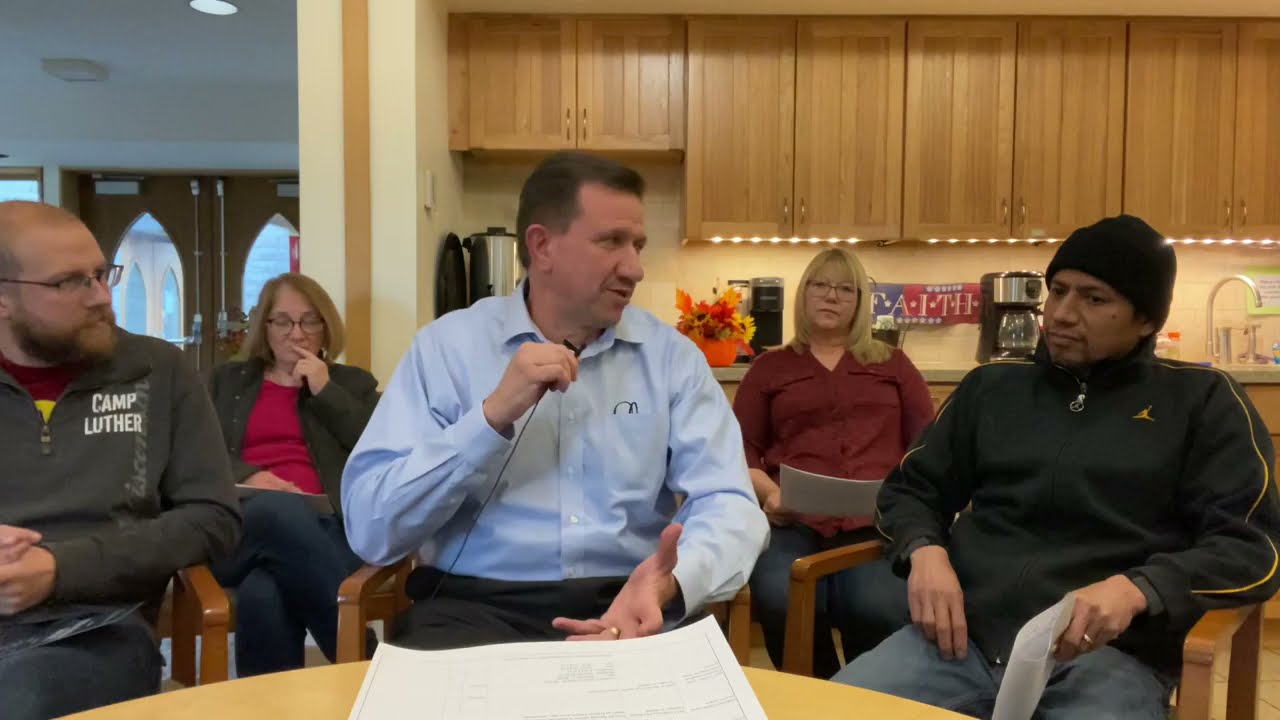This image captures a detailed scene of a small group discussion taking place in a room that resembles a kitchen area within a church, characterized by its background architecture and decor. The horizontally aligned rectangular picture shows five people focused on a central conversation. Prominently in the center, a middle-aged man dressed in a blue collared button-down shirt holds a small microphone, suggesting he may be leading the discussion. Flanking him on his right side (our left), a man in a gray button-down shirt bearing the name "Camp Luther," with glasses, brown facial hair, and a shaved head, appears engaged. To the central man's left (our right), another man, dressed in a black beanie, a black and yellow striped jacket, and jeans, sits pensively. 

In the background, on either side of the central man, sit two women with short blonde hair, dressed casually, contributing to the casual, community atmosphere of the room. The setting includes cabinets, a sink, and a banner near a coffee maker that reads "Faith," reinforcing the assumption that this is part of a church. Additional details include double doors with large windows in the upper left corner, through which more light filters, enhancing the setting’s clarity and depth. The image as a whole encapsulates a moment of collective focus and communication, possibly revolving around a community or church-related activity.